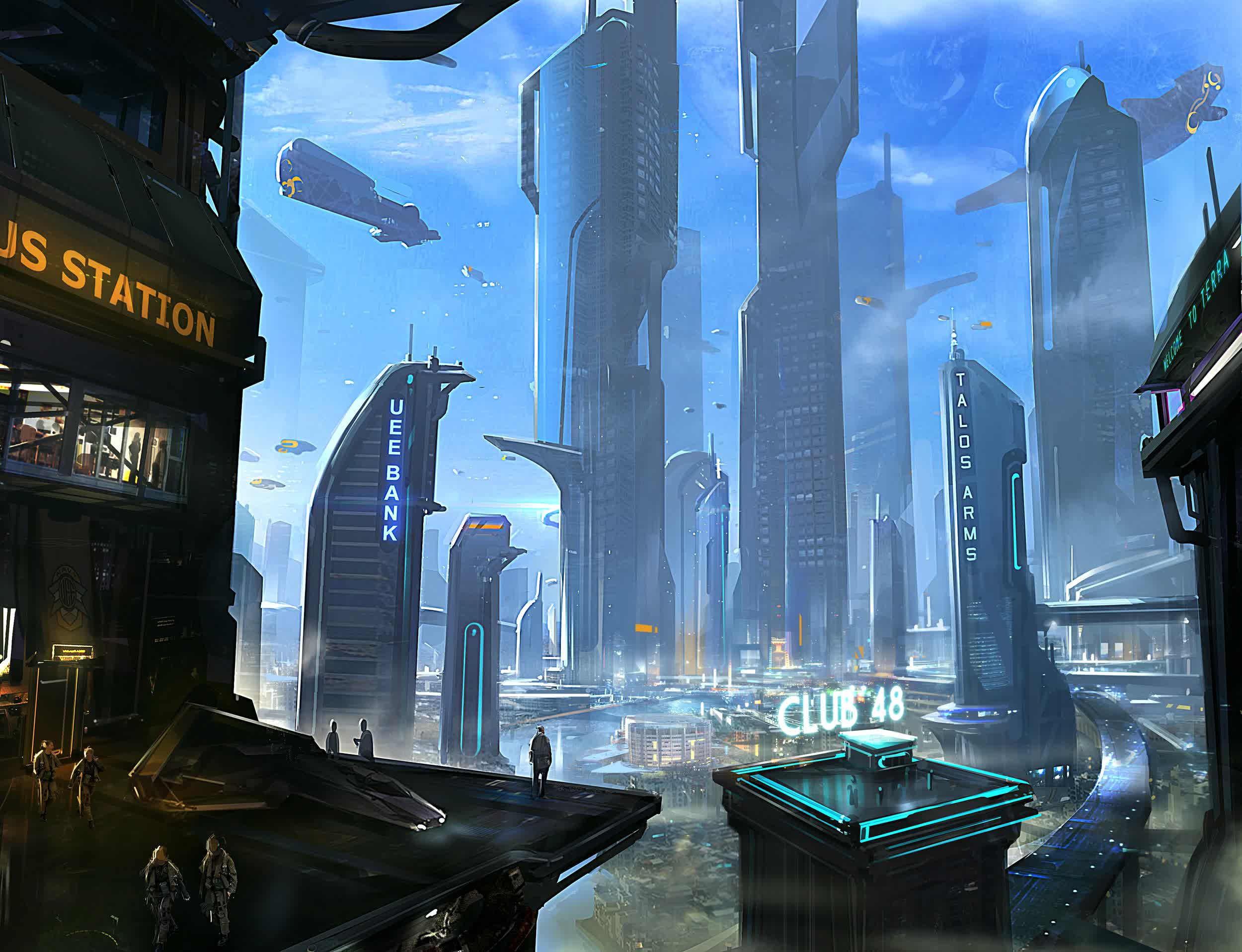This is a highly detailed, computer-generated illustration of a futuristic city, possibly out of a science fiction novel or video game. The cityscape features an intricate mix of towering, abstractly shaped skyscrapers adorned with neon lights in hues of blue, black, and aqua. Amidst the skyline, large dirigible-looking ships and smaller, car-sized hover vehicles crisscross the bright blue sky, illuminated by the sun.

In the background, notable buildings include the "UEE Bank" and "Talos Arms," both labeled in striking blue text. The "Club 48" sign, set against a building with glowing aqua roof lights, stands out prominently in the mid-distance. On the left side of the image, a structure marked "US Station" (with part of the sign obscured) functions as a busy hub. Tan-uniformed people mill around a sophisticated-looking flying vehicle parked on an elevated platform at the station, as if preparing for takeoff.

Additionally, a hint of a secondary planet appears faintly behind the high-rises. The lower part of the city appears submerged in water, possibly remnants of an older city now lying beneath the futuristic metropolis. The illustration seamlessly blends elements of high-tech futurism with a post-apocalyptic atmosphere, creating a vivid and immersive urban scene.